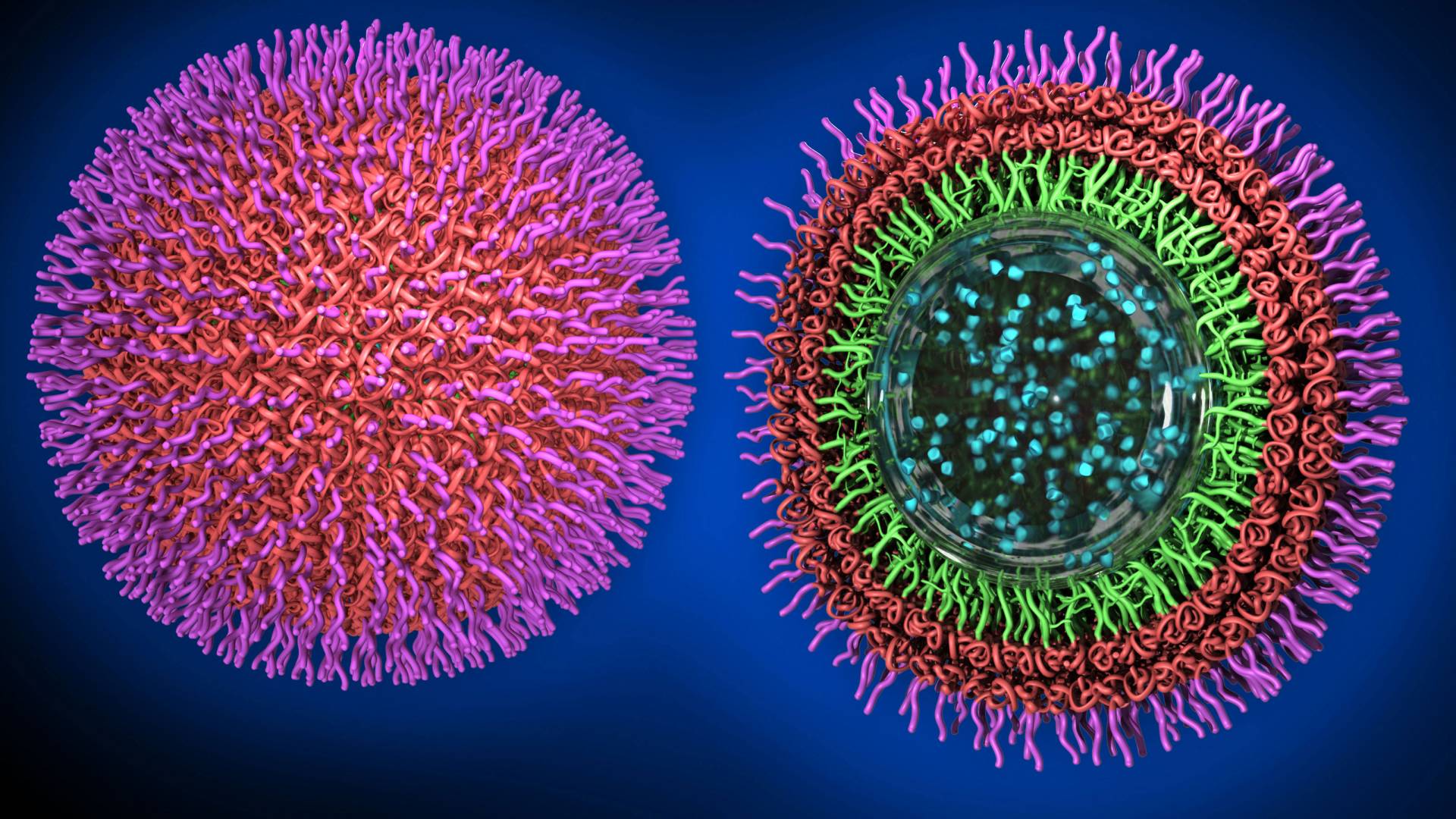The image features a blue background framing a blackish-blue rectangle, emphasizing a striking contrast. On the left side, there's a spiky, ball-shaped object resembling a flower, predominantly orange at its core with short, hair-like antennas radiating outwards in a violet-lavender hue. This composition of the object creates a visually captivating burst of color from its orange base. To the right, an image details what appears to be a cross-section of this spiky ball. The cross-section reveals a black center dotted with glowing aqua blue specks. Surrounding the center are concentric rings of spines; the innermost layer is green, followed by orange, and finally violet-purple spikes radiating outwards, creating a layered, eye-catching pattern. Overall, the image presents a fascinating study in contrasting colors and intricate textures.